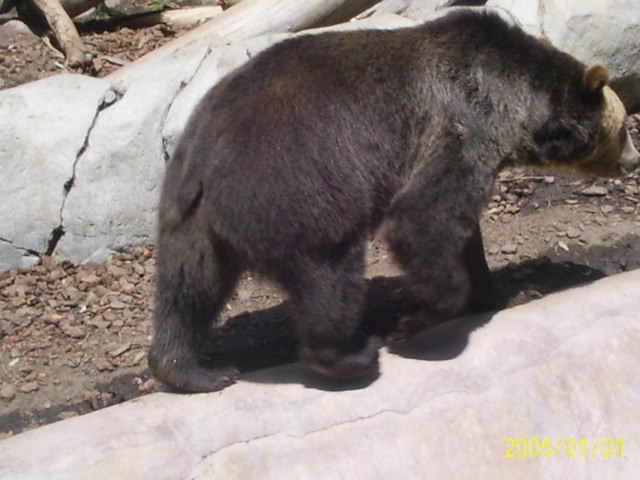This is a detailed wide rectangular photograph of a black bear walking along a cement enclosure, possibly at a zoo, dated 2005-01-01 in yellow text at the bottom right corner. The bear's body is covered in black fur with a cream-colored face, and it has a small tail. It’s in a walking position with its right front leg lifted and right back leg slightly hovering above the ground, casting a clear shadow on the stony and soil-covered ground. The image captures a side view of the bear from left to right, with its head in the top right corner and its backside towards the center left. The ground includes areas covered in tiny gray and reddish-brown rocks. There is a smooth, light gray ledge running diagonally from the bottom left to the middle right of the image. Behind the bear lies a taller, smooth gray rock and white stones, creating the backdrop. Additionally, brown logs and wood chips are scattered on the ground, enhancing the naturalistic setting of the bear’s environment during the day.